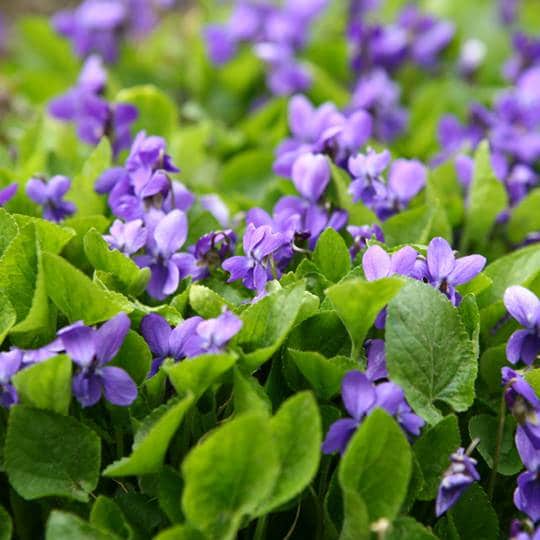This photograph captures a densely packed field of vibrant greenery and small purple flowers. The lush green leaves, prominently veined, dominate the lower portion of the squared image, gradually blurring towards the top. Among these leaves, delicate purple flowers with four to five petals each emerge, creating a striking contrast. The blossoms range in shades from light to dark purple, with some clusters catching more light, particularly in the background, giving a nuanced play of illumination across the scene. The flowers, featuring oval petals around a small center, create a consistent, atmospheric overlay of purple atop the green. This detailed, layered portrayal showcases both the intricate beauty of each individual flower and the overwhelming abundance of nature as it stretches into a slightly out-of-focus distance.